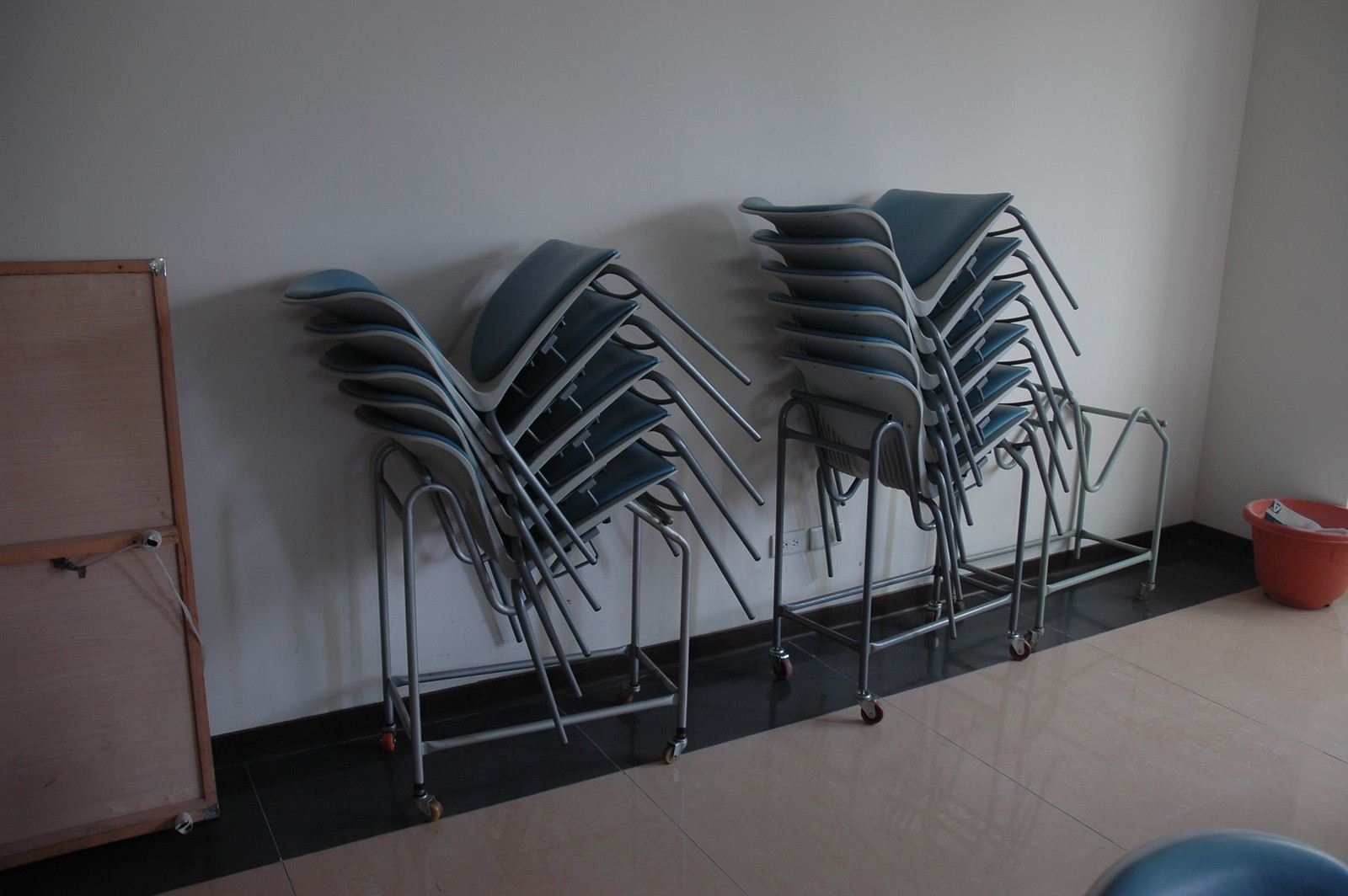The image captures the interior of a room with a plain white wall in the background. Situated against the wall are two stacks of chairs, each with padded backrests and seats, placed on angled steel frame racks equipped with wheels. Next to these two filled racks, there is an empty frame, also with wheels. The chairs, which may be typically found in schools or public buildings, have a slight backward tilt hinting at imperfect stacking. They feature a bluish color and four metal silver legs. To the right side of the room, there is a large red bucket or pot with some items inside. To the left of the stacked chairs, there appears to be a wooden bowling table backed up against the wall. The floor is a light-colored tile that reflects some light, with black edging around the perimeter of the room. A blue ball can also be observed in a corner near the wooden bowling table.